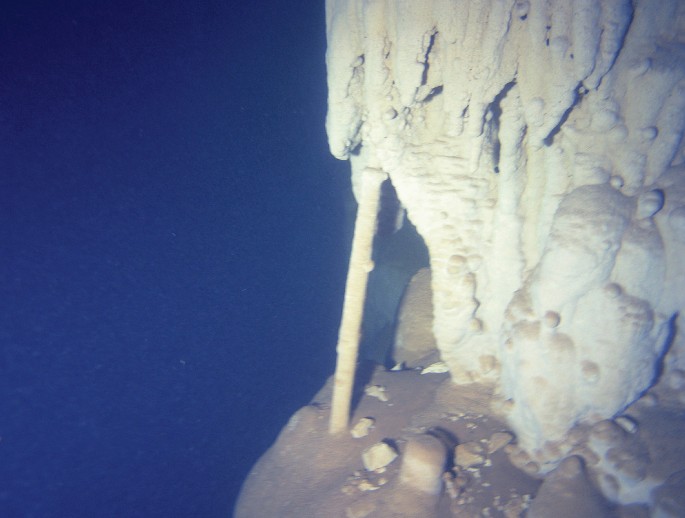This underwater photograph, likely taken in the ocean, captures a mysterious and intriguing formation. The right side of the image is dominated by what appears to be a coral-like structure, with a blend of white, light brown, and creamy wax-like textures. This formation, possibly resembling an underwater mountain or volcano, features a metal drum at its base, from which a pipe extends upward, further covered by this waxy buildup. The edges of this formation exhibit shades of yellowish color, adding to its intricate appearance. The backdrop on the left side of the photo presents a sea of dark, empty blue water, with no visible wildlife, enhancing the enigmatic and solitary nature of the scene. Scattered around the bottom, dark brown pieces that resemble shrapnel or debris contribute to the complexity of this underwater landscape.